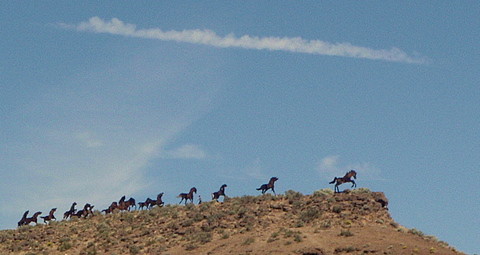In this outdoor photograph, a side view captures a group of wild horses galloping across a slight incline on a hill. The scene is set against a backdrop of a blue sky that transitions from a darker hue at the top to a lighter shade near the horizon. A thin, white cloud stretches horizontally about an inch from the top of the image, accompanied by faint, wispy clouds dispersed throughout. At the horizon on the left, a bright light suggests the presence of the sun from that direction, enhancing the natural illumination of the scene. The hill itself, covered primarily in dirt with sparse greenery and desert-like brush, rises gently before tapering off near the right edge of the image with a small drop-off. The horses, predominantly dark-colored and slightly out of focus due to the distance, are seen in various stages of their stride, some with their hooves off the ground. Most of the horses are clustered together towards the right, with a few stragglers nearing the edge of the drop-off, all heads uniformly facing and moving towards the right.